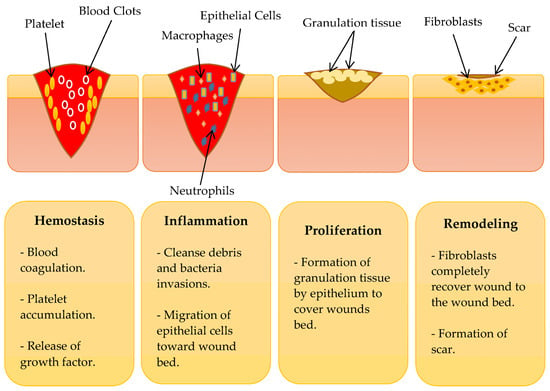This diagram illustrates the stages of skin healing with a sequence of four images and corresponding labels. 

The first image depicts the epidermis and dermis layers with red and yellow circular shapes representing blood clots and platelets. This stage is labeled "Hemostasis," indicating blood coagulation, platelet accumulation, and the release of growth factors.

In the second image, rectangular yellow shapes represent macrophages, while rectangular blue shapes represent epithelial cells. This stage is labeled "Inflammation" and emphasizes cleaning debris, bacteria invasion, and the migration of epithelial cells towards the wound bed.

Moving to the third image, the epidermis and dermis contain granulation tissue depicted by a smaller, cream-colored triangle. The label beneath this image is "Proliferation," focusing on the formation of granulation tissue by epithelial cells to cover the wound bed.

The fourth and final image shows the skin with fibroblasts and scar formation, indicated by red circles with yellow outlines. This stage is labeled "Remodeling," highlighting the role of fibroblasts in completely covering the wound bed and forming a scar.

The bottom part of the diagram provides additional notes and terms related to each stage, reinforcing the processes of hemostasis, inflammation, proliferation, and remodeling in skin healing.